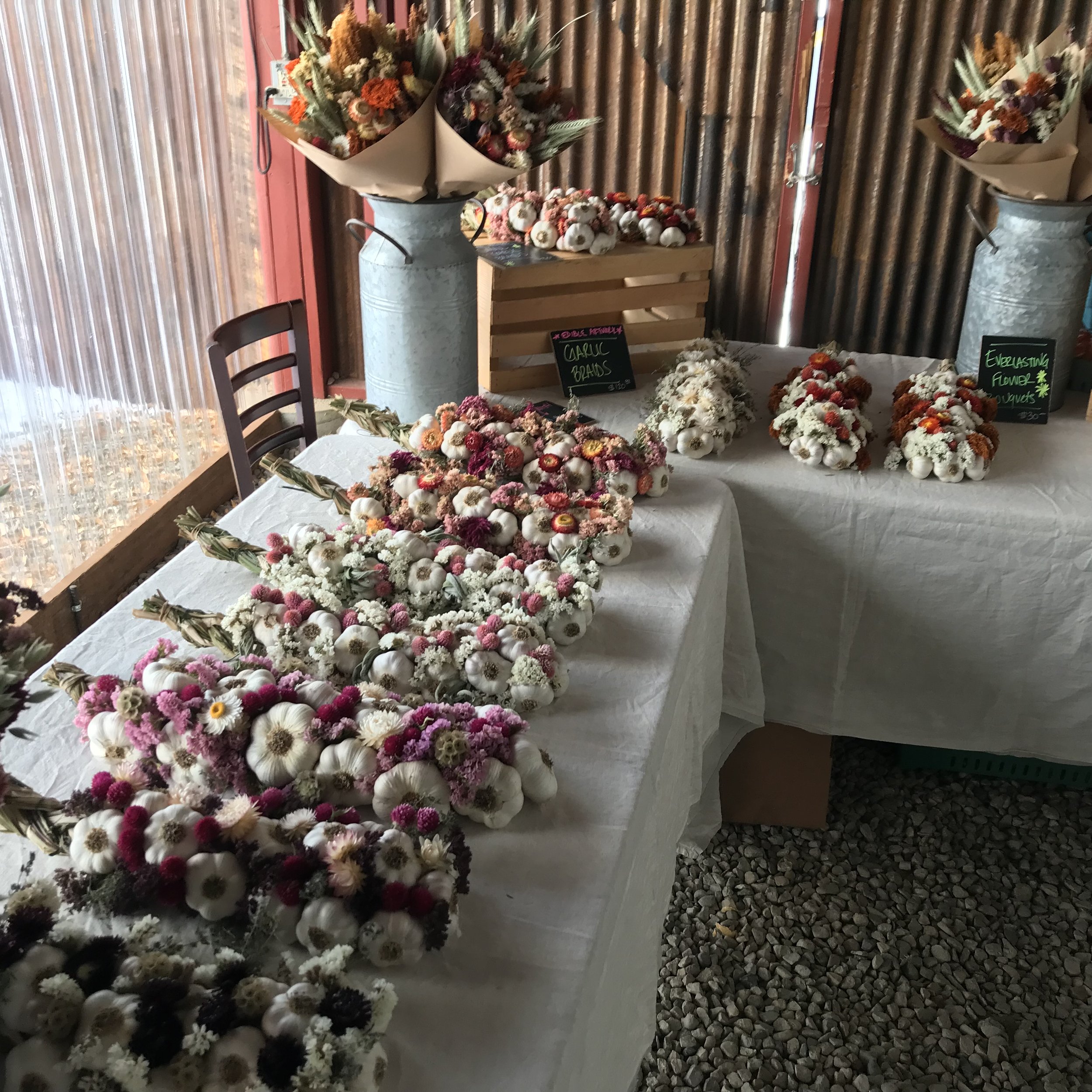The image displays a quaint arrangement of two tables positioned perpendicularly, each draped with pristine white linens. The floor beneath features a layer of gray pebbles. One wooden chair is stationed at the intersection of the tables. Adorning these tables are several bouquets, specifically seven on one and three on the other, with colorful blossoms in shades of cream, purple, red, light pink, magenta, yellow, and dark orange. Intermingled with the flowers are whole garlic bulbs and braids, wrapped in natural, cardboard-colored paper. Each table also holds a large metal flower pot brimming with additional floral arrangements. Behind this elegant setup stands a metal gate, adding a rustic touch to the scene. Signage includes a chalkboard labeled "garlic braids" and another sign reading "everlasting flower." This scene, encapsulated within what appears to be an indoor area with steel walls, evokes a charming blend of natural beauty and rustic elegance.